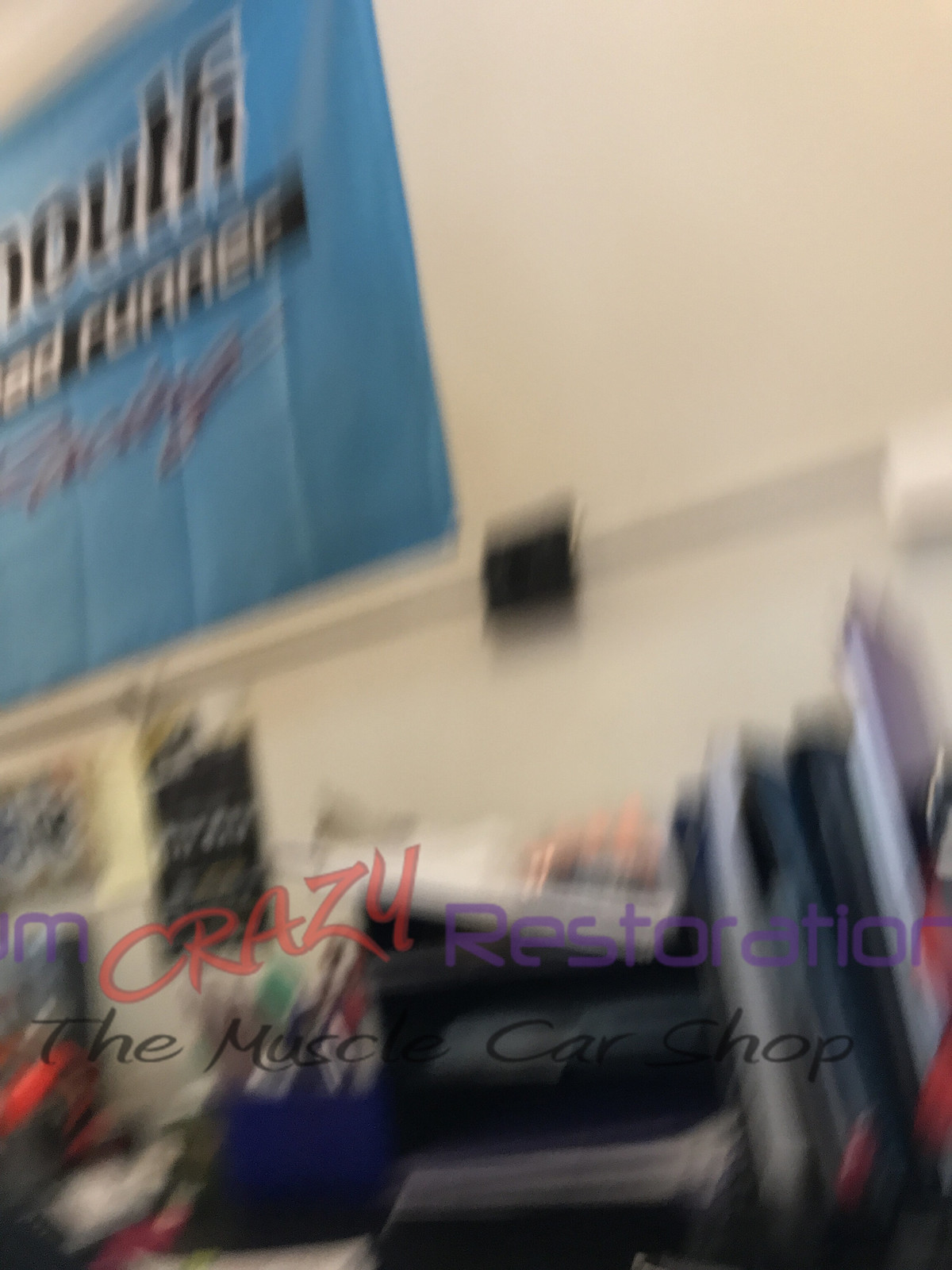The image is a blurred photograph of an indoor setting, likely taken vertically with a cell phone. Dominating the scene are several prominent text elements and signs. In the foreground, the words "crazy," written in bold red capital letters, "restoration," in purple, and "the muscle car shop," in black, are clearly visible, suggesting the image is watermarked by a business named "Crazy Restoration Muscle Car Shop." On the left, there is a distinctive purple symbol. The background features what appear to be books and retail merchandise, although the heavy blurring makes it difficult to discern specific details. The wall is primarily white, and on the top left, there is a blue border or sign with the partial text "ad runner" and "youth" in black letters, with additional text in red cursive underneath, though it is not entirely readable. A small black object is also visible at the bottom of the image.